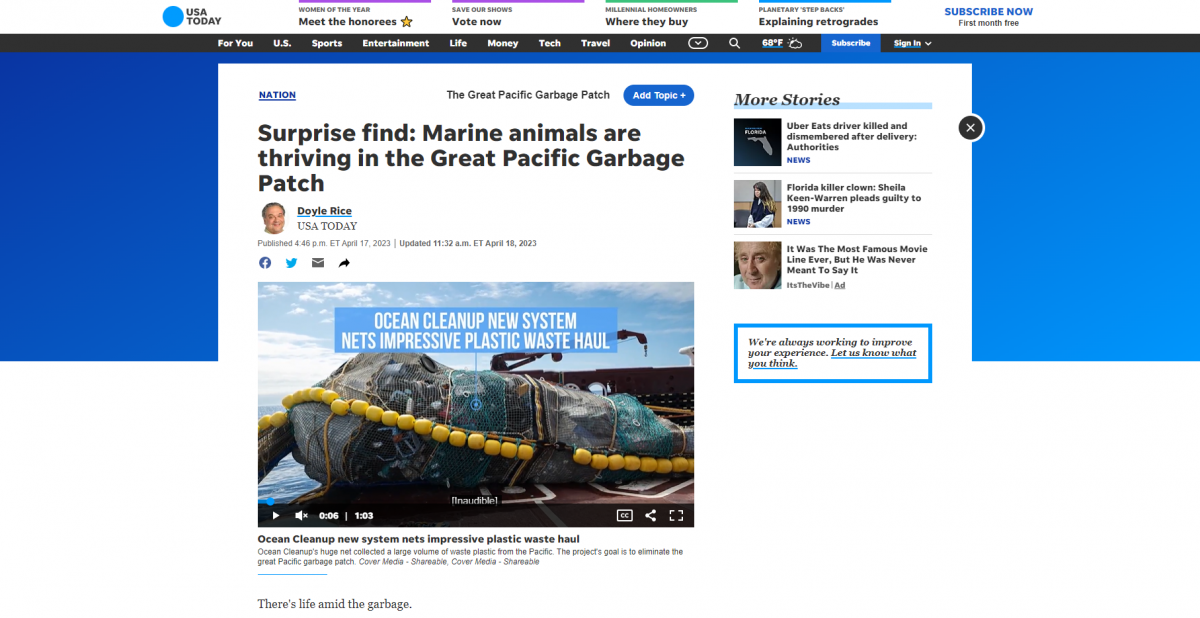This screenshot from USAToday.com features a detailed and color-coded navigation menu located at the top of the page. The options provided include "Women of the Year," "Meet the Honorees," "Save Our Shows," "Vote Now," "Millennial Home Owners," "Where to Buy," "Planetary Stepbacks," a partially unreadable option, "Explaining Retrogrades," and "Subscribe Now." 

To the left of these options, the prominently recognizable USA Today logo can be seen. The main menu, distinguished with bars above each item in colors purple, green, and blue, includes categories such as "For You," "US," "Sports," "Entertainment," "Life," "Money," "Tech," "Travel," "Opinion," as well as search functionalities, and options to "Subscribe" or "Sign In." The "Subscribe" option is visually emphasized with a blue highlight, indicating it is either selected or prompted for user action.

Dominating the central view is a white panel headlined "Great Pacific Garbage Patch," accompanied by a feature to "Add this topic." The article, authored by Doyle Rice, details a surprising discovery: Marine animals thriving in the Great Pacific Garbage Patch. An image within the article shows garbage being extracted by nets, with the caption "Ocean Cleanup, New System Nets Impressive Plastic Waste Hauls."

Adjacent to this main feature, the sidebar to the right lists additional stories. These include topics related to Florida, a case involving a "Florida Clown Killer," and what appears to be a reference to the movie "Willy Wonka." Beneath this segment, there's a blue rectangle containing a brief blurb, hinting at further content.